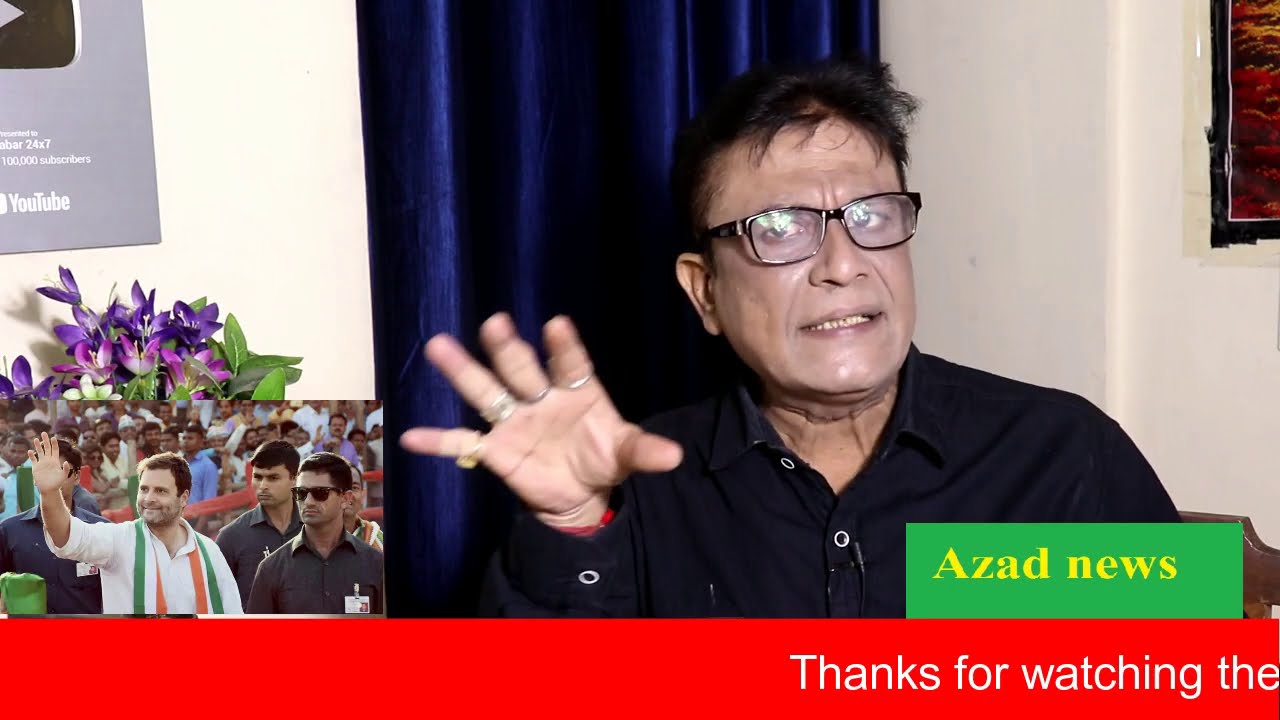In this detailed image, a man with short, mangly black hair and black-rimmed glasses is the focal point. He's holding out his right hand, prominently displaying silver rings on all his fingers except his thumb; his pinky is wrapped in a bandage. He's wearing a black button-up shirt with white buttons. His mouth is open, showing his top teeth.

To the man’s left is a dark blue curtain, while to his right is a white wall partly covered by a black-edged painting of a turbaned man with dark brown skin. Below this, on the bottom right corner of the image, there's a green banner with "Azad News" in yellow text. Below that stretches a red banner with "Thanks for Watching" on the right side and a silver YouTube play button, signifying 100,000 subscribers, on the left. Just below this is an image or video still that the man seems to be reacting to, showing a crowd of people. In this image, one man in a white shirt with green, white, and red stripes on his scarf holds his hand up. Beside him are two security guard-like figures in black outfits, with the rightmost individual wearing black sunglasses. Purple and pink flowers are placed right beneath this display.